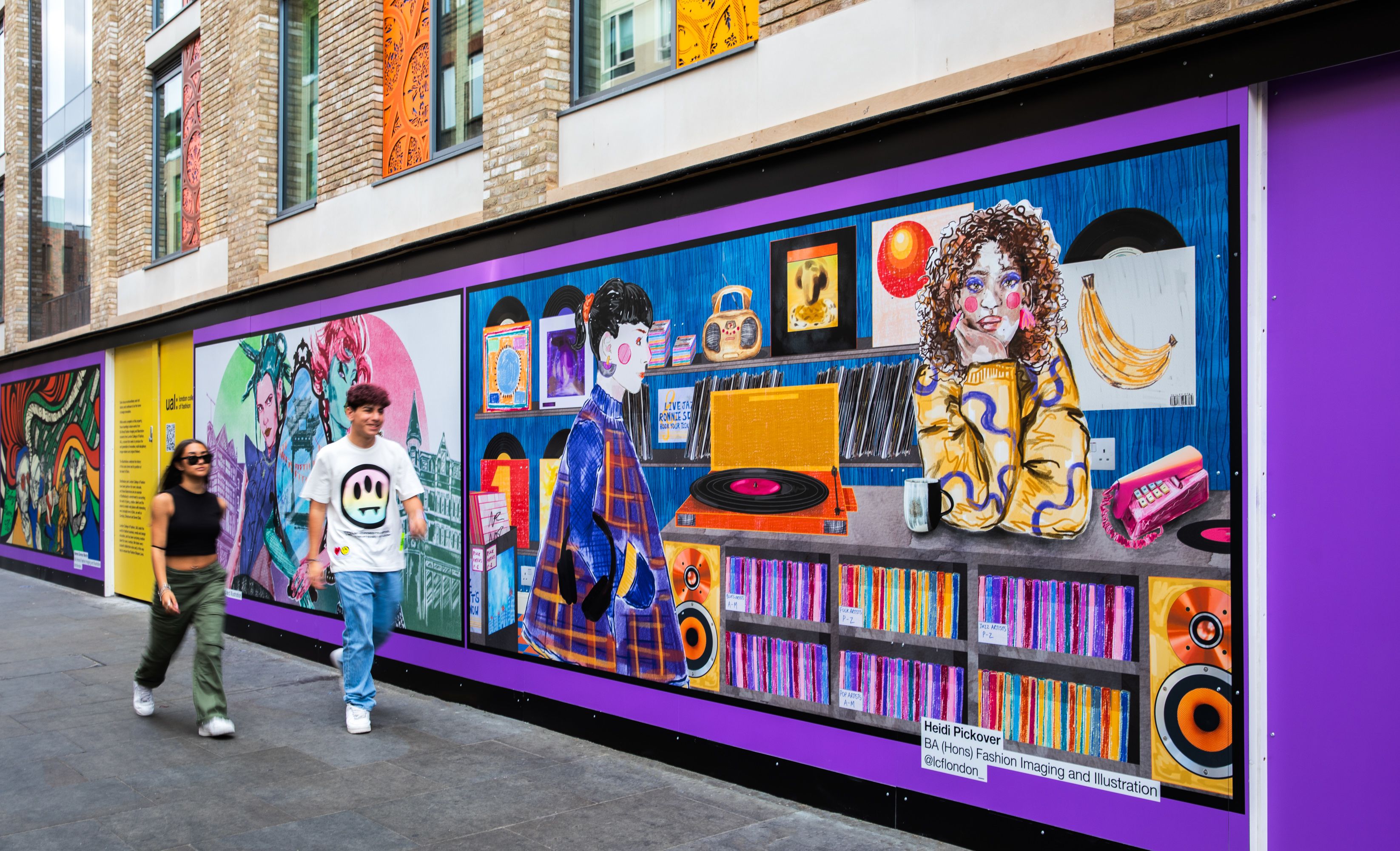The photograph captures a vibrant street scene where two individuals stroll past a detailed mural on the side of a brick building. The woman wears green army-style pants, a sleeveless black top, white sneakers, and sports sunglasses with her black hair cascading down. Beside her, the man dons a white t-shirt emblazoned with a unique smiley face featuring vampire teeth and three eyes in pink, yellow, and blue hues, paired with blue jeans and white sneakers. 

The mural they walk past is rich in detail, featuring a scene from a nostalgic record store. It showcases a girl leaning on a counter with her elbow propped up and her chin resting in her palm, as if deep in thought. This main artwork is surrounded by depictions of a record player spinning a black vinyl record, an array of colorful album covers including one with a banana and another orange-hued one, and a classic boombox. The mural bears the name "Heidi Pickover, B.A. Hans, Fashion Imaging and Illustration at LCF London," framed within a purple border. Above the mural, windows punctuate the brick façade of the building, completing this urban tableau.